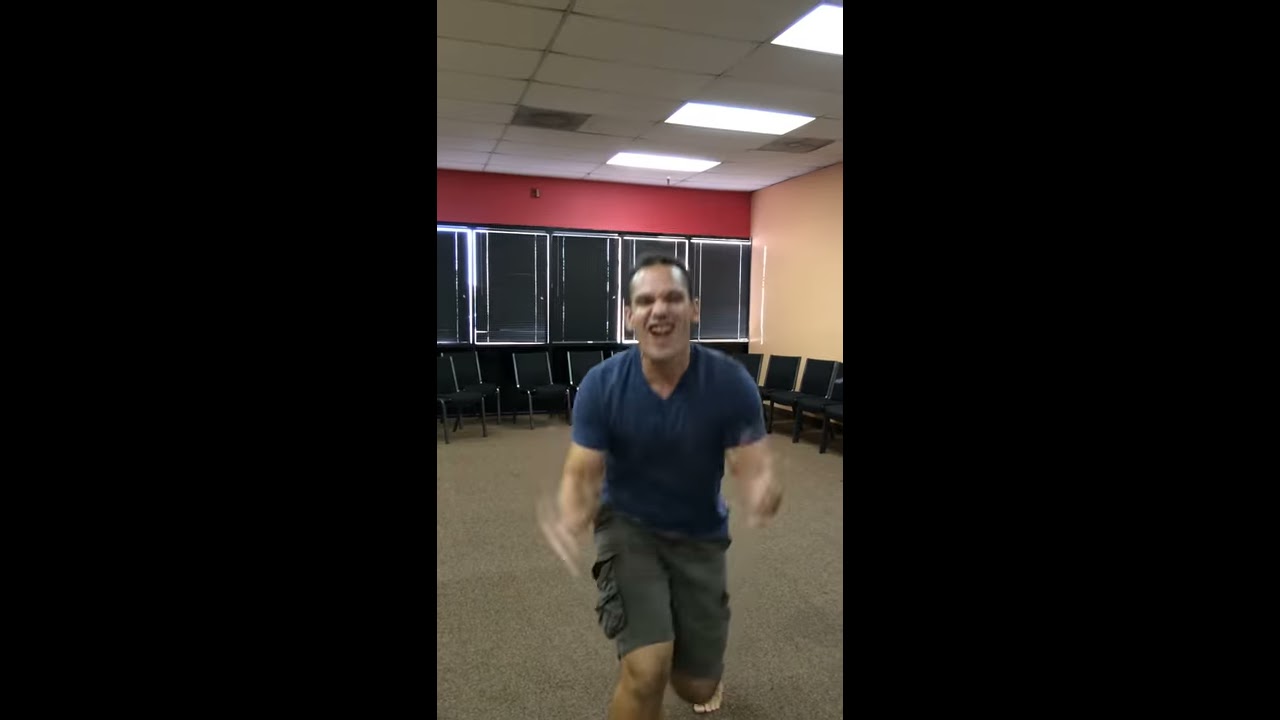The image captures a young man energetically posing in a room, wearing a blue t-shirt and light gray khaki shorts. He is barefoot, with his body leaning forward in a lunge towards the camera, adding a dynamic blur to his hands. His face is scrunched up into a broad smile, showing his front top teeth. The background features brown industrial carpeting and a semi-circle of black metal chairs stretching from the left to the right. Behind him, an orange wall transitions into a red strip above a series of windows covered with black blinds, allowing some light to filter through. Overhead, the ceiling is composed of white panels with inset lighting, while an orange wall is noticeable on the right side.